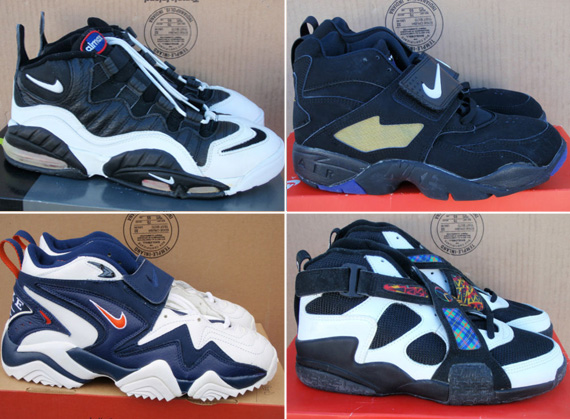This image showcases a neatly arranged collection of four pairs of children's Nike sneakers, each pair occupying its own quadrant within the divided frame. 

In the top left section, there is a pair of black and white Nike sneakers featuring white laces and also velcro fastenings. They are positioned prominently with a shoe box visible in the background, adding context and depth to the display.

The top right quadrant displays another pair of Nike sneakers, predominantly black with subtle white accents, complemented by a large velcro buckle on the front. The accompanying box in the background further emphasizes the brand identity.

Shifting to the bottom left, a pair of white and black Nike sneakers with a striking red swoosh stands out. These sneakers also have their box visible, showing various stamps and informational text, enhancing the visual appeal.

Lastly, the bottom right quadrant presents a pair of mostly white sneakers adorned with intricate crisscross straps in red and blue. This pair diverges slightly in style, lacking the Nike swoosh but maintaining a dynamic and decorative appearance. The background similarly features a shoe box, tying together the cohesive theme of branded footwear.

The overall presentation, combining detailed brand logos, vibrant color contrasts, and visible packaging, suggests a meticulously crafted product photo, possibly intended for resale on platforms like eBay.